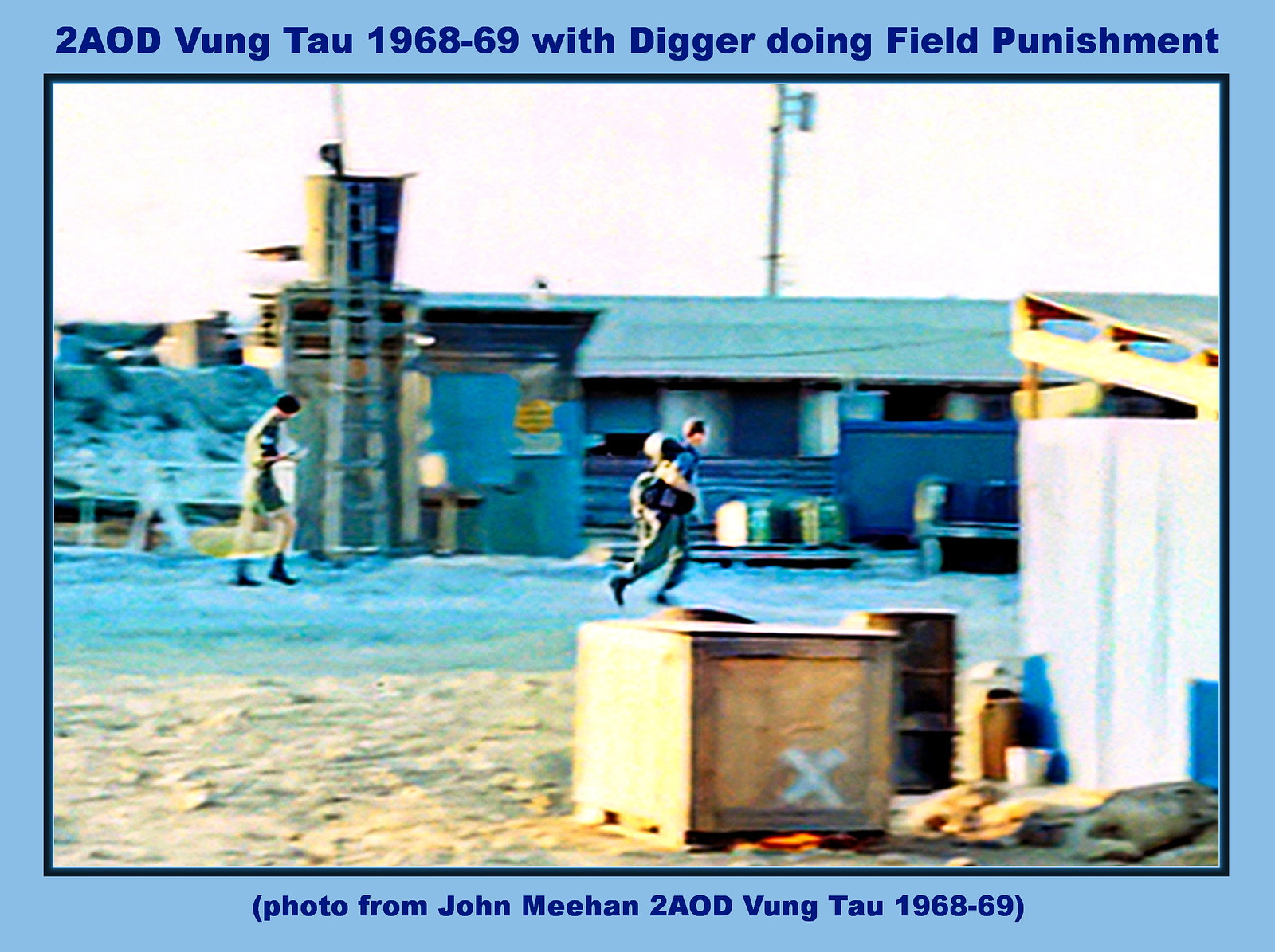This photograph, annotated with blue text at the top and bottom, captures an outdoor scene at a military base in Vung Tau, Vietnam, during 1968-69. The top text reads "2AOD Vung Thao 1968-69 with Digger doing field punishment," and the bottom text states, "Photo from John Meehan 2AOD Vung Thao 1968-69." The image features a pair of men, presumed soldiers, one walking and the other in a running position, wearing equipment strapped to their bodies. Background structures include several buildings, and in the foreground, a large wooden box marked with a white "X," an oil drum, and possibly a wooden shed can be seen. Despite the image's blurriness, it vividly portrays a snapshot of military life and field activities during the Vietnam War.